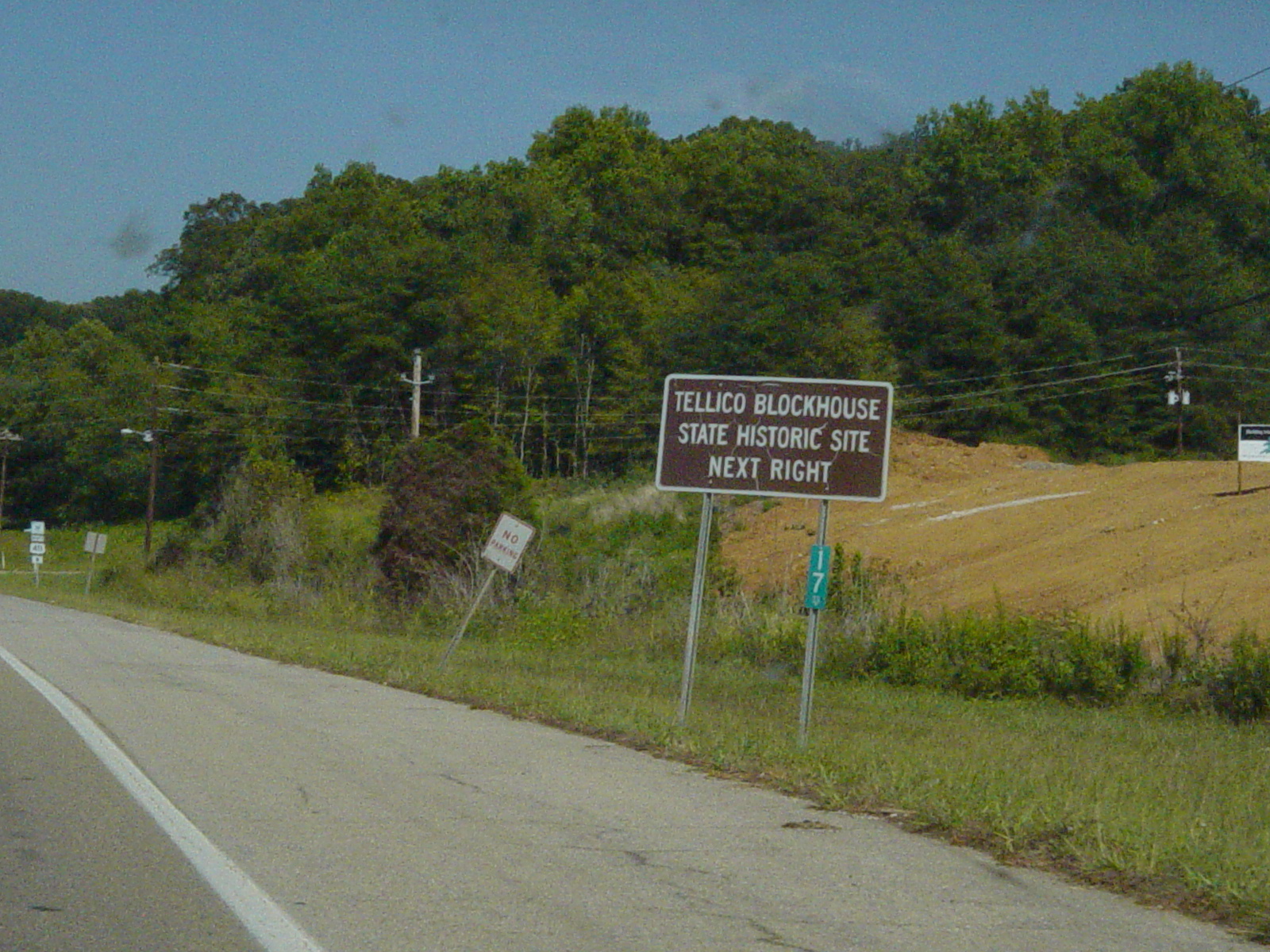In this daytime photograph, we see a detailed landscape showcasing a highway scene dominated by a road sign. The sky above is a vibrant blue with scattered clouds, suggesting fair weather. Positioned along the right shoulder of the highway, the road sign stands out with its brown background and white border, clearly displaying the message "Tellico Blockhouse State Historic Site Next Right" in white lettering. Beneath this directive, a green mile marker marked "17" is visible. Surrounding the sign, the immediate area transitions from grassy patches to a dirt section, hinting at possible construction activity. Further in the background, the landscape is framed by a concentration of trees, with several above-ground power lines crossing in front, adding to the depth and complexity of the scene. The edge of the photograph hints at additional signage at the construction site, but it is partially out of frame. This well-composed image captures the essence of a highway moment leading to a historic site, set against a tranquil yet active environment.